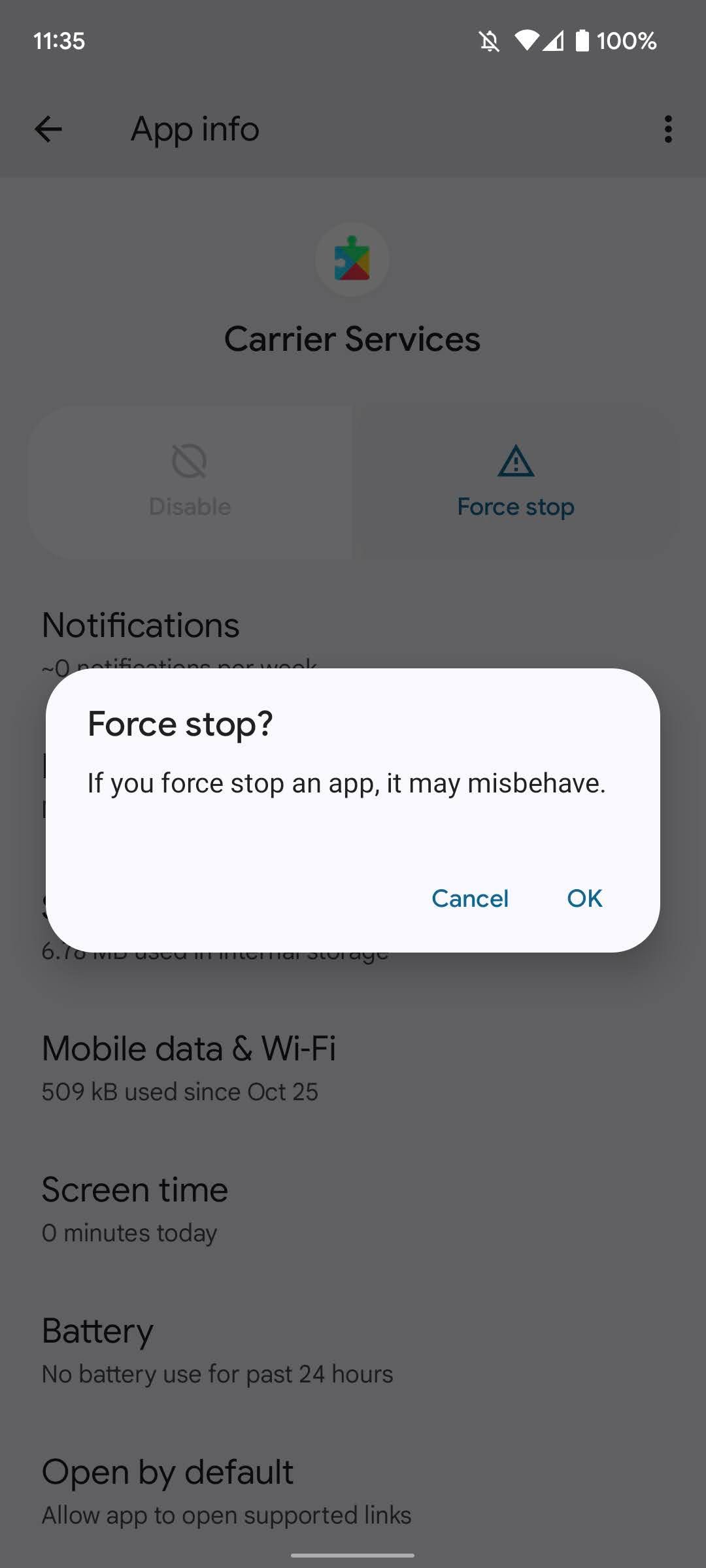This screenshot captures a moment within the settings of a smartphone, showcasing the App Info screen specifically for the "Carrier Services" application. The status bar at the top displays the current time as 11:35, a fully charged battery at 100%, strong WiFi connection, muted sound, and three-quarters cellular signal strength.

The user is contemplating a force stop of the "Carrier Services" app. This is evident from the visible pop-up window that warns, "If you force stop an app, it may misbehave," and provides two options: "Cancel" and "OK." The main screen beneath the pop-up reveals further details about the app: the notifications management section, data usage (509 kilobytes since October 25th), screen time (zero minutes per day), battery usage (no usage in the past 24 hours), and default app opening behavior (allowing the app to open supported links).

The imminent action from the user—whether to cancel or confirm the force stop—is anticipated but not yet determined. The setting provides a clear view into the app's minimal impact on system resources, adding context to the user’s decision to force stop the application.